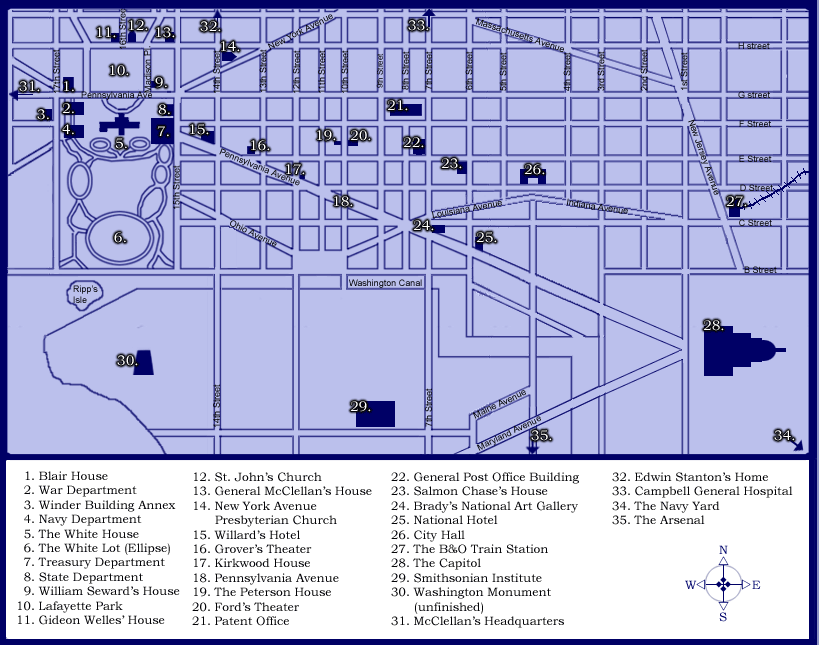This image is a detailed map bordered in dark purple with a light purple background. It features an extensive list of numbered locations, which correspond to various buildings and landmarks as outlined in the legend below the map. The map also includes a compass in the bottom right-hand corner, showcasing directions: north, south, east, and west. 

Highlighted locations on the map include prominent government and historical sites such as:

1. Blair House
2. War Department
3. Winter Building Annex 
4. Navy Department
5. The White House
6. The White House Ellipse
7. Treasury Department
8. State Department
9. William Seward's House
10. Lafayette Park
11. Gideon Wells House
12. St. John's Church
13. General McClellan's House
14. New York Avenue Presbyterian Church
15. Willard's Hotel
16. Grover's Theater
17. Kirkwood House
18. Pennsylvania Avenue
19. The Peterson House
20. Ford's Theater
21. Patent Office
22. General Post Office Building
23. Salmon Chase's House
24. Brady's National Art Gallery
25. National Hotel
26. City Hall
27. B&O Train Station
28. The Capitol
29. Smithsonian Institute
30. Washington Monument (unfinished)
31. McClellan's Headquarters
32. Edwin Stanton's House
33. Campbell's General Hospital
34. The Navy Yard
35. The Arsenal

The map indicates significant government buildings, historical homes, churches, theaters, and other important landmarks, providing a comprehensive guide to the area it covers.